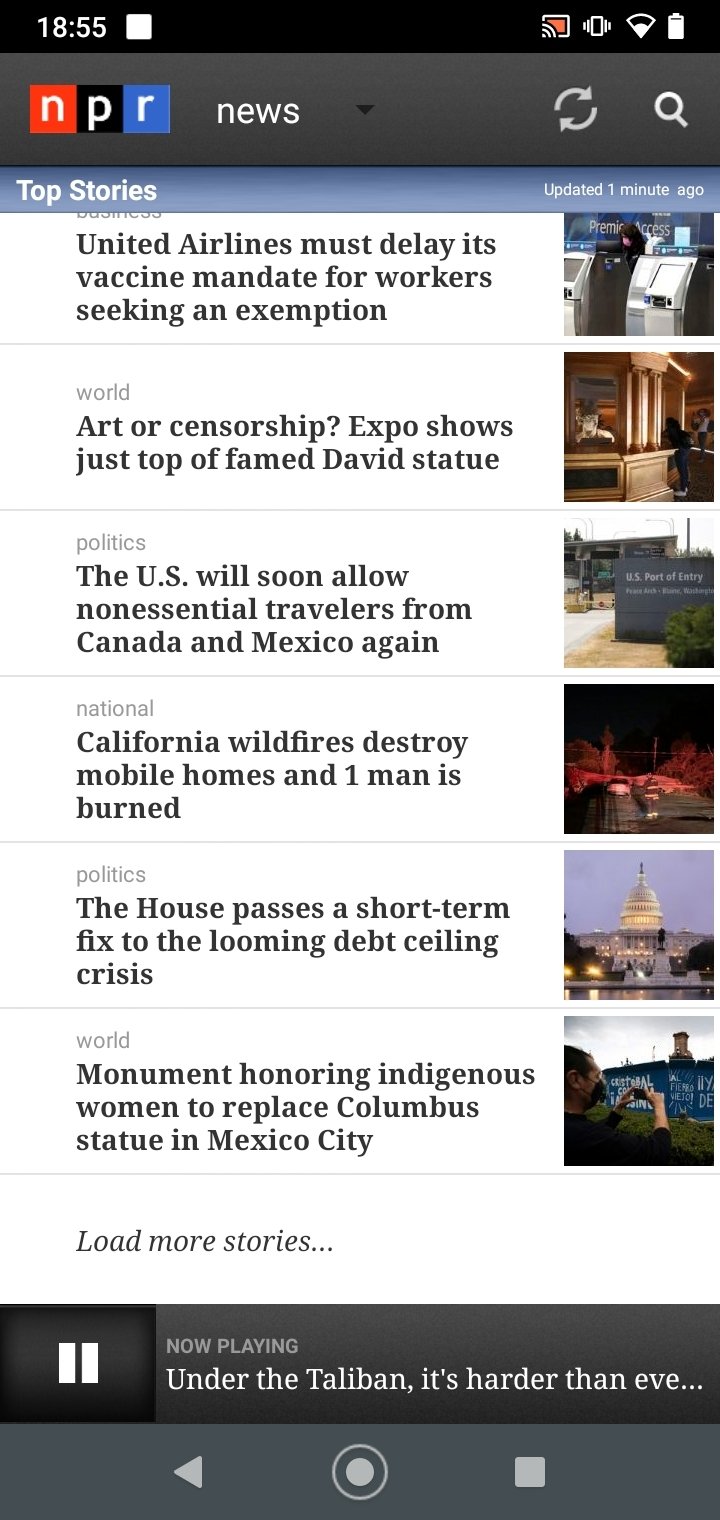This image captures the screen of a tablet or iPhone, identified by its aspect ratio and the visible status indicators at the top, which show the time as 18:55, battery level, wireless connectivity, and vibration mode. Just below these indicators, a black bar prominently displays the words "News" and "NPR," accompanied by icons for search and refresh functionalities.

Beneath this bar is a section titled "Top Stories," presenting a list of current articles. The highlighted stories include:

- An article on United Airlines delaying its vaccine mandate for workers seeking exemptions.
- A feature titled "Art or Censorship?" discussing an expo showcasing the top of the famed David statue.
- News about the U.S. allowing non-essential travelers from Canada and Mexico again.
- Coverage of California wildfires that have destroyed mobile homes and resulted in one man being burned.
- A report on the House passing a short-term fix to the looming debt ceiling crisis.
- An article about a monument honoring indigenous women that will replace the Columbus statue in Mexico City.

At the screen's bottom is another black bar, which features the caption "Now playing under the Taliban, it's harder than ever," next to a large pause button. The very bottom of the image includes the standard navigation icons typical of an Android device.